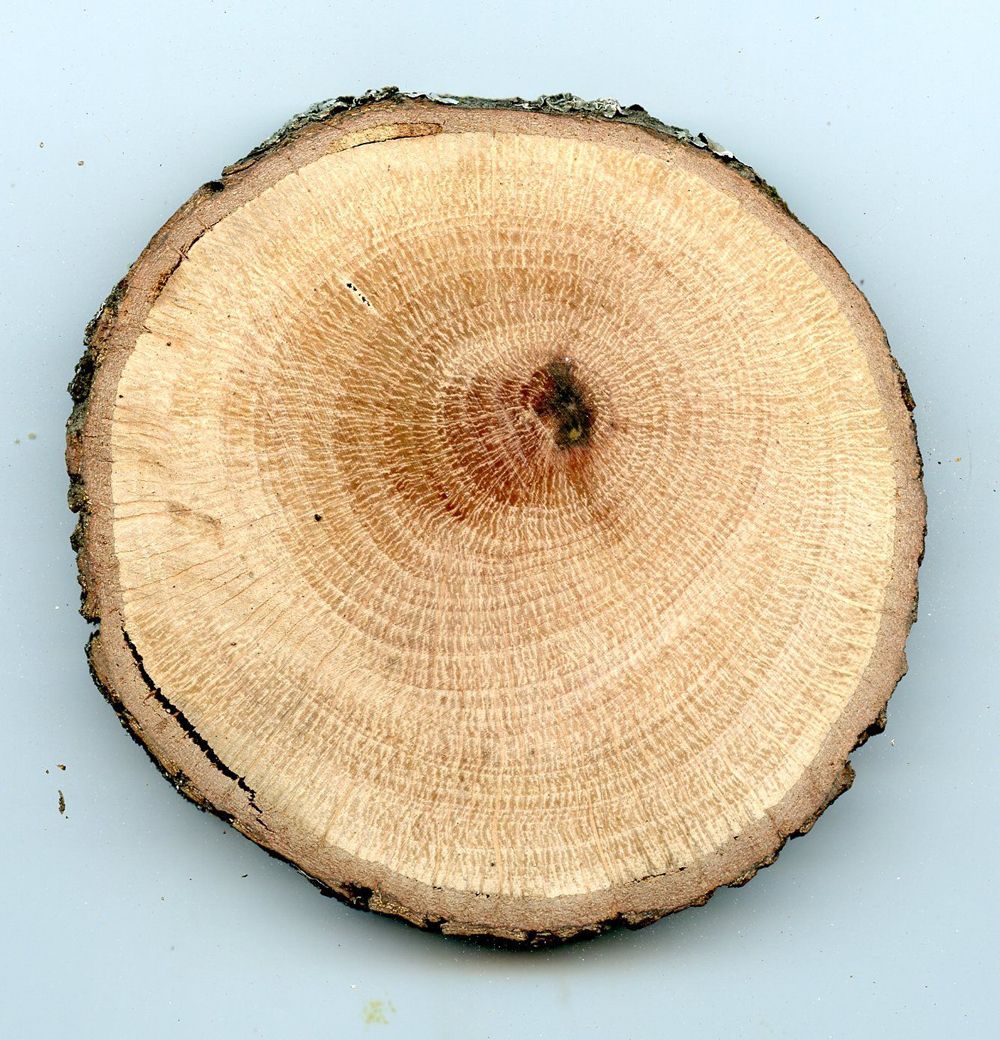This photo showcases a detailed top-down view of a cut tree trunk slice, prominently displayed against a smooth turquoise blue background. The round cross-section reveals intricate wood grain patterns, with numerous concentric rings marking the tree's age. The bark encircles the outer edge, appearing as a blend of brown, dark gray, and hints of green moss, suggesting it might be a pine or cedar. The wood inside starts light brown, darkening progressively towards the center, where it features a reddish-brown hue and a slightly charred or burnt-looking spot, indicative of the cutting process. The overall image captures the raw, unrefined beauty of natural wood, with the fine details of the tree's life history etched into its rings.